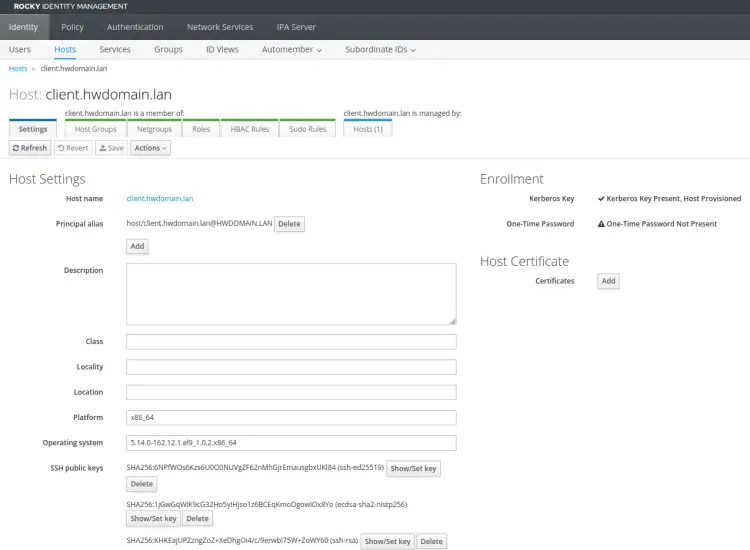The screenshot showcases the Rocky Identity Management interface, specifically focusing on the "Hosts" page within the "Identity" tab. At the top, five clickable tabs are visible: Identity, Policy, Authentication, Network Services, and IPA Server. The "Identity" tab is currently selected, revealing additional categories such as Users, Hosts, Services, Groups, ID Views, Auto Member, and Subordinate IDs, with the "Hosts" category highlighted in blue.

The main section of the interface displays detailed host-related management options. It identifies a particular host as Host.Client.HWDomain.LAN, with this host marked as managed. A set of navigation tabs including Settings, Host Groups, Net Groups, Roles, HBAC Rules, Pseudo Rules, and Hosts (1) are present beneath the host's identification.

Below the navigation tabs, a form titled "Host Settings" appears, inviting the user to fill in various fields. These fields include Host Name, Principal, Alias, Description, Class, Locality, Location, Platform, and Operating System. Users can interact with the form using buttons labeled Refresh, Revert, Save, and Actions, facilitating modifications and updates to the host's information.